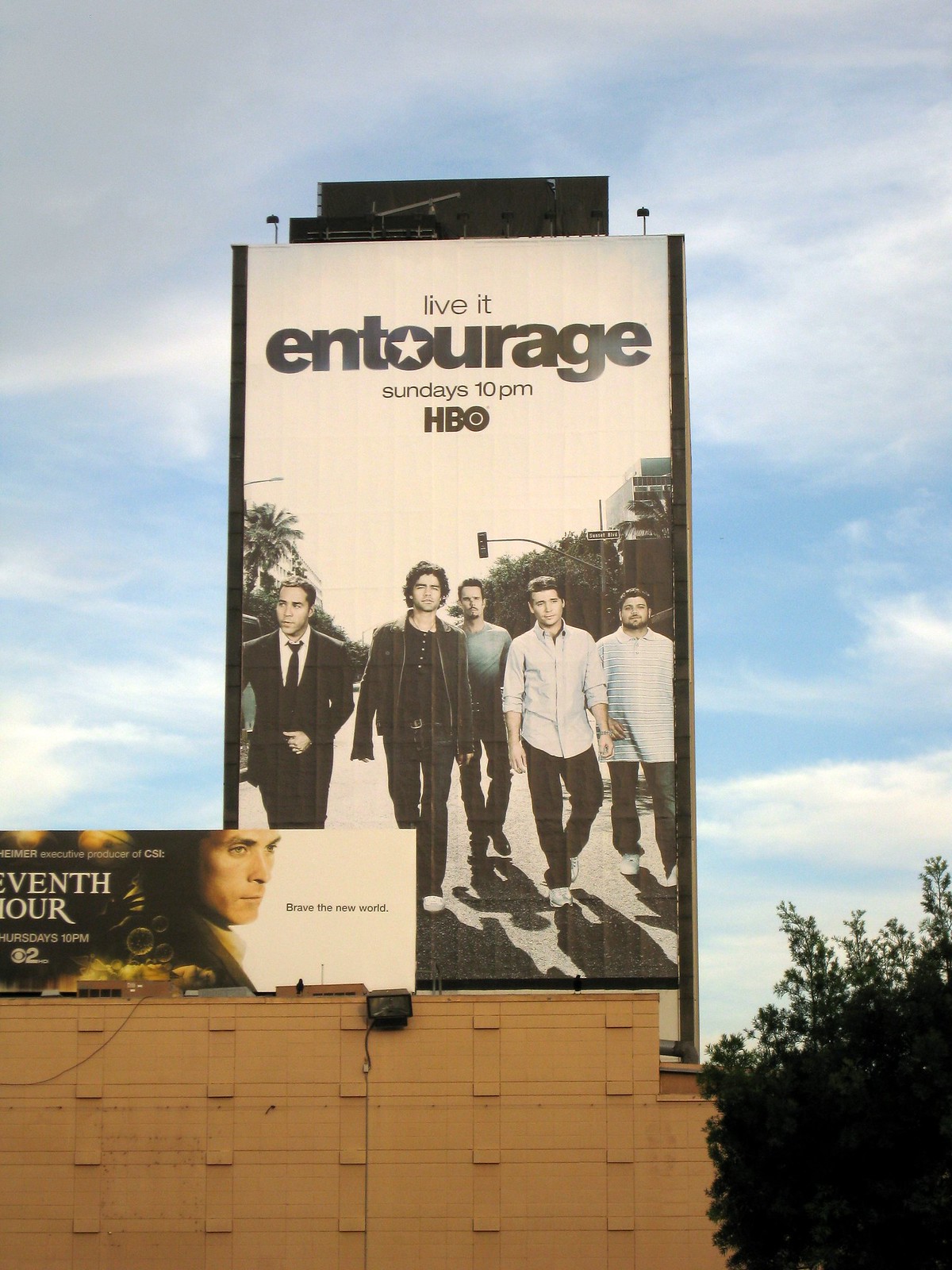The photograph captures an outdoor scene featuring two prominent billboards mounted on the rooftop of a brown brick building against a backdrop of a blue sky with hazy clouds. The larger, portrait-oriented billboard advertises the HBO show "Entourage," emblazoned with the tagline "Live It" and the air time "Sundays 10 p.m." The billboard's background is predominantly white, with a dramatic image of five young men walking toward the viewer along a tree-lined street, their figures backlit to create dark shadows in front of them. The characters are dressed in casual attire, with one distinctly wearing a suit and tie. Behind them, a faint traffic light is visible. 

To the left of this large advertisement is a smaller, horizontal billboard for "7th Hour." This sign also features a white background with black text stating "Brave the New World," and showcases a pensive man's face in profile. The building supporting the billboards is partially visible and appears orange-beige in some areas. In the lower right corner of the image, a bush is spotted, adding a touch of greenery to the urban setting. The billboards are equipped with spotlights at the top, suggesting they are well-lit during nighttime.